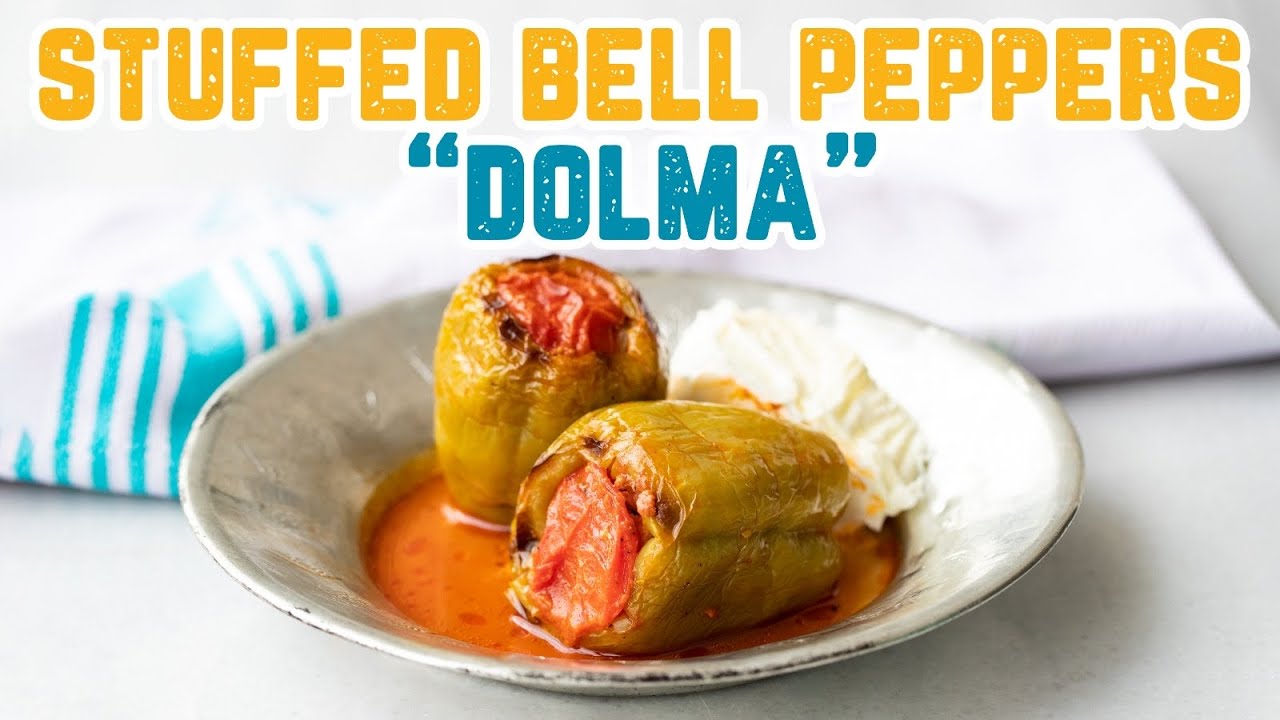This is a detailed photograph, possibly a screen capture from a video or presentation, showcasing a dish of stuffed bell peppers, labeled at the top with "STUFFED BELL PEPPERS” in all caps yellow font, and “dolma” in blue-green font, both framed in white. The image features a small white bowl containing a single green bell pepper split in half and stuffed with a mixture that includes rice and tomatoes. The stuffed peppers appear slightly charred and are sitting in a red tomato-based sauce, with a dollop of sour cream alongside. The bowl rests on a smooth white surface, with a white tablecloth or dish towel with blue stripes visible in the background, adding a touch of color to the setting. The overall composition makes the dish look quite appetizing.